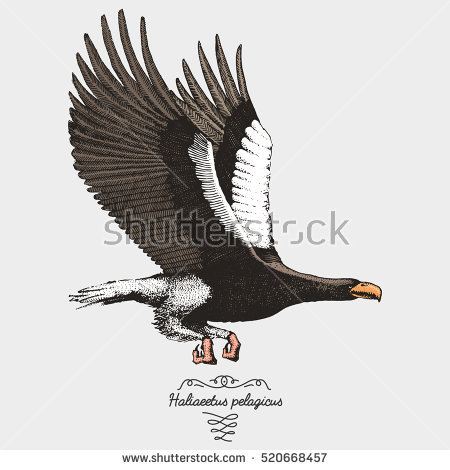The image shows a bird, likely an eagle, in mid-flight with a large wingspan set against a gray background. The bird features gray feathers with white tips and has a distinctive yellow beak. Its feet, adorned with orange claws, are visible towards the bottom. The wings exhibit a pattern with rows of white, black, and gray feathers. On the left side of the bird, more white feathers can be noted. The bottom of the image displays the text "Haliaeetus pelagicus," the scientific name for the bird, along with "www.shutterstock.com" and the image number "520-668-457." A Shutterstock watermark is overlayed on the image, which appears to be an illustration.